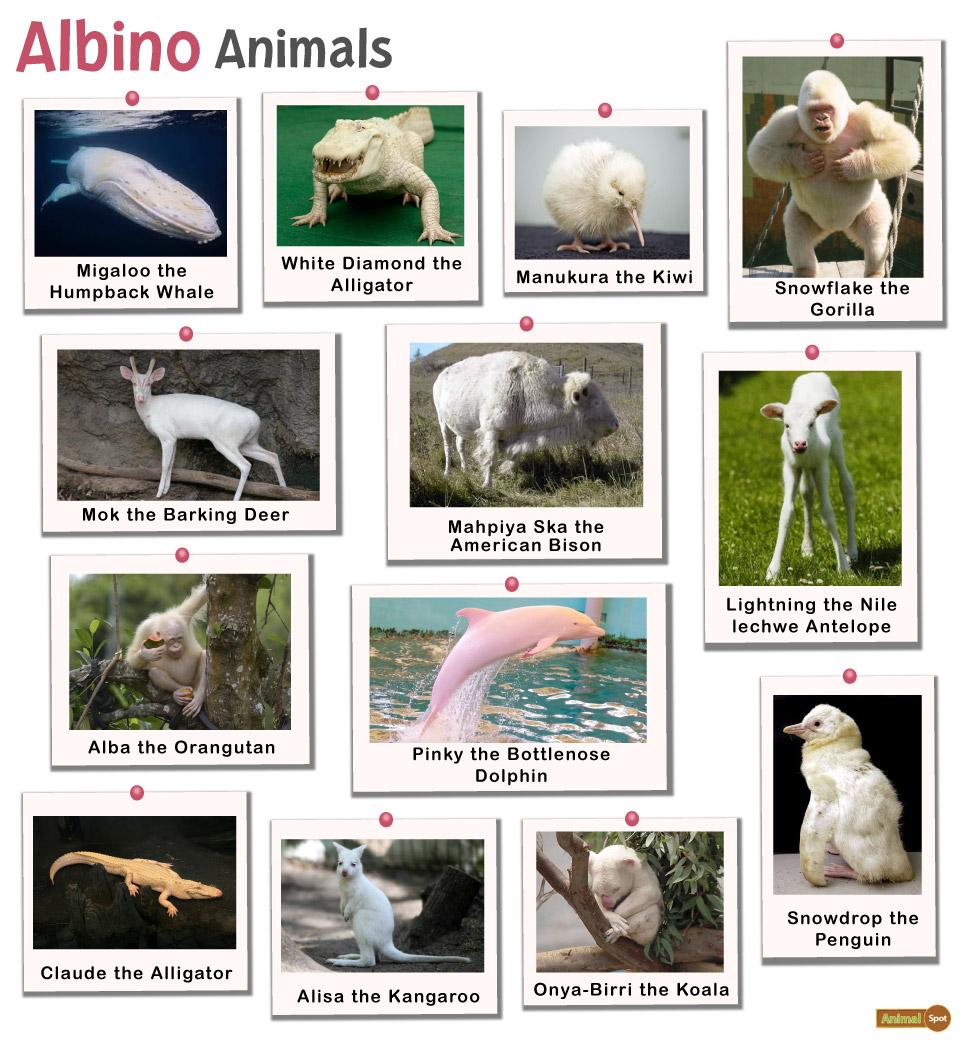This image showcases a collection of twelve photographs, each depicting a unique albino animal, arranged in an orderly grid on a white background. At the top center, the bold red title "Albino" is followed by "Animals" in black letters. Each photograph is bordered by a small note card with the animal's name, tacked with red pins for a digital scrapbook effect. Starting from the upper left, the photos include:

1. Migaloo, the humpback whale, featuring a white whale swimming.
2. White Diamond, the alligator, showing a whitish-yellow alligator.
3. Manukuru, the kiwi, portraying a light-colored chick.
4. Snowflake, the gorilla, displaying a standing albino gorilla.
5. Mock, the barking deer, with a white deer shown in profile.
6. Mapayaska, the American bison, with a side view of a grayish bison.
7. Lightning, the Nile lechwe antelope, showing a young antelope standing outside.
8. Alba, the orangutan, featuring a light gray orangutan in a tree.
9. Pinky, the bottlenose dolphin, displaying a pink dolphin leaping from water.
10. Claude, another alligator, with a small, light yellow alligator against a black background.
11. Elisa, the kangaroo, featuring a small white kangaroo in profile.
12. Anyabiri, the koala, showing a small animal on a tree branch.

In the bottom right corner, a logo in orange, white, and green reads "Animal Spot." This gallery of rare albino animals emphasizes their unique and striking appearances, showcasing their white coats and skin tones in a compelling visual display.